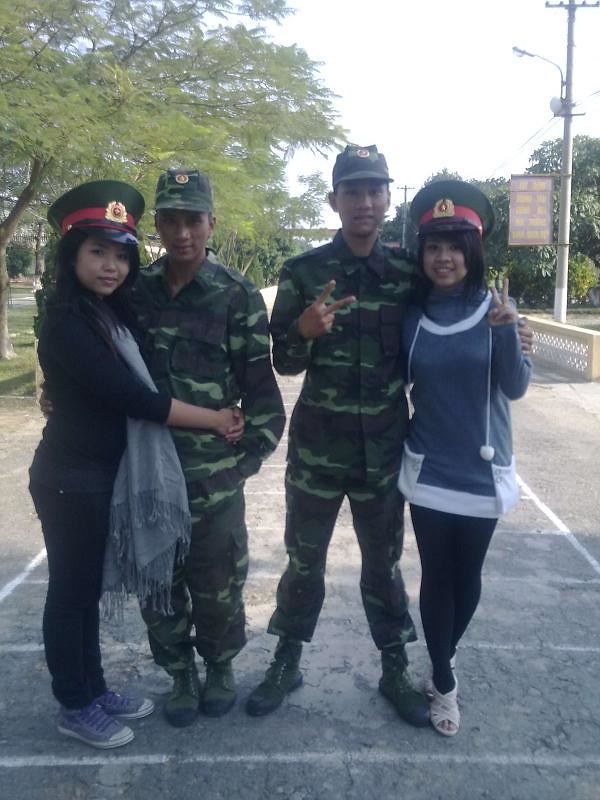In this vibrant outdoor scene, four people, consisting of two couples, stand confidently in a crosswalk against a backdrop of urban elements including buildings, trees, and power lines. The couple on the right features a woman with shoulder-length dark black hair, dressed in a gray top with white rings around the collar and thighs, black pants, and cream-colored sandals. She strikes a peace sign with one hand while her other hand wraps around a man beside her, the tallest individual in the group, clad in a camouflage suit with matching boots and hat, also wearing a gold and red emblem on the hat. His left arm is also holding up a peace sign. To their left stands another man, similarly dressed in a camouflage outfit and hat, with one hand in his pocket and his other arm around the woman beside him. The woman on the far left, facing to the right but looking back at the camera, sports curly black hair flowing down her back, a gray top with a badge, a scarf transitioning from black to gray, a black long-sleeve shirt, black pants, and purple shoes. The scene is anchored by a detailed crosswalk painted white on an asphalt surface, juxtaposed with a bright tree adorned with green lights on the left and a utility pole with a street light and a sign on the right. The sky behind them is a stark white, contributing to the overall color palette of blacks, grays, greens, and touches of gold and red.